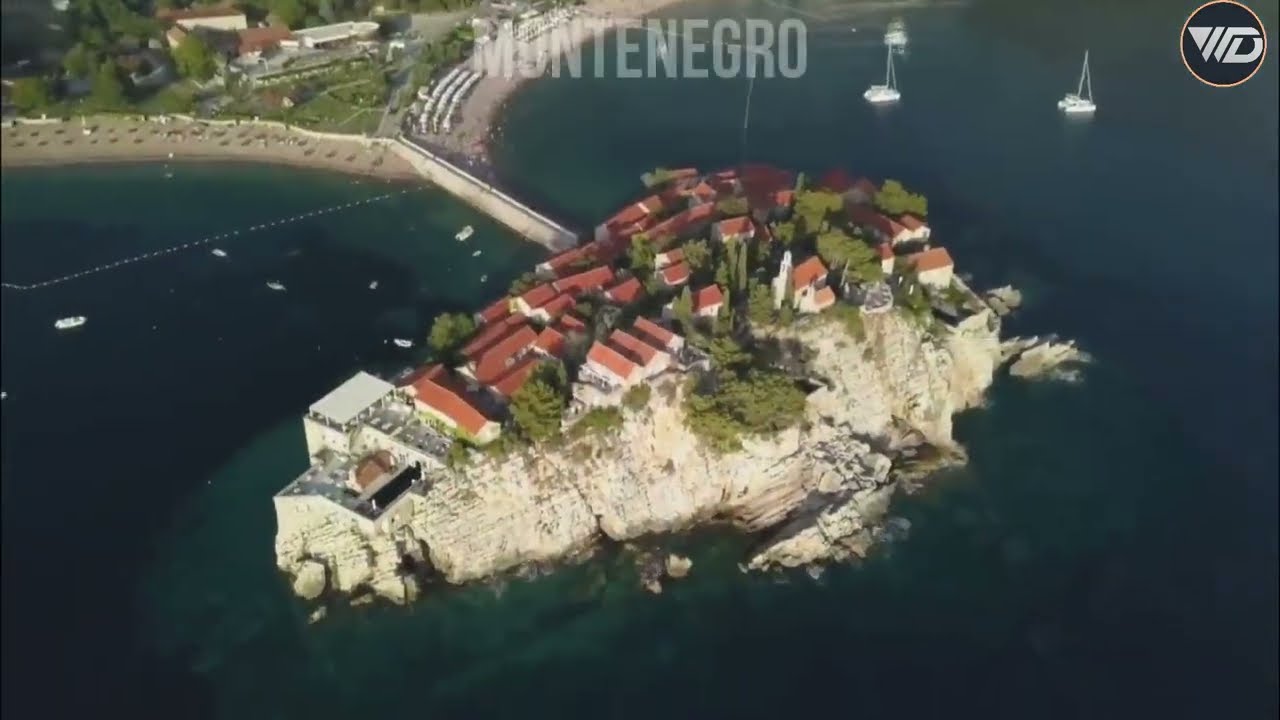The image presents an aerial view of a compact, rocky island prominently placed in the center. The island is distinguished by its steep, white stone cliffs adorned with dense green foliage. The landscape is densely packed with numerous rectangular structures, featuring red clay roofs that contrast with the lush greenery. Jutting from the island towards the upper left corner of the image is a narrow cement bridge, connecting to a nearby shoreline. This adjacent land displays more red-roofed buildings and a verdant expanse of grass and trees, alongside a beach shore. Surrounding the island is a vast body of deep blue water, populated by several white sailboats. The setting is bathed in daylight, indicating an outdoor scene. At the top of the image, the word "Montenegro" is written in transparent lettering, accompanied by a logo in the top right corner.